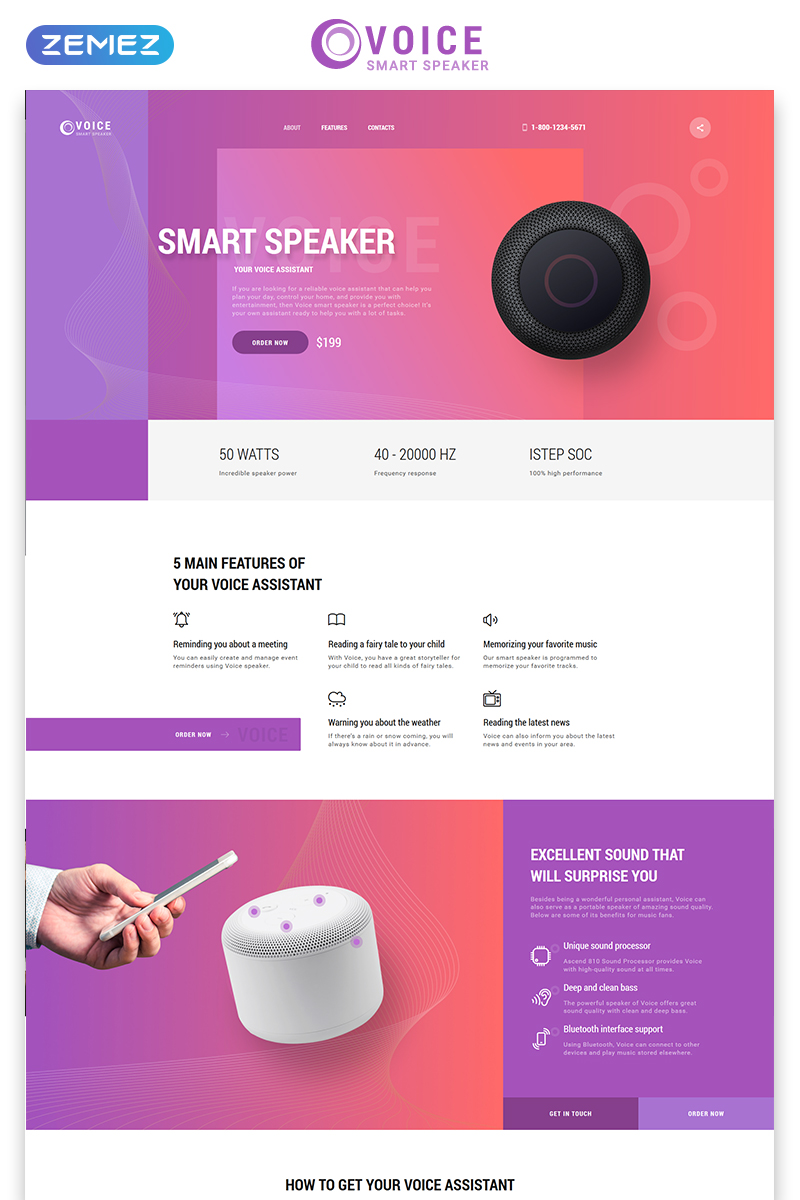The website for Zmez showcases a sleek and modern design, prominently featuring a rounded rectangle or pill-shaped graphic with a blue-purple gradient background. The name "ZMEZ" is displayed twice in bold white text. Central to the homepage is a purple logo on a white background, coupled with the text "Voice Smart Speaker" in a clean, legible font.

The layout is visually striking, utilizing a mix of purple and pink gradients to create an engaging aesthetic. At the top, header text boldly announces "Smart Speaker," accompanied by an image of the speaker itself. A call-to-action invites users to "Order Now" for $199.

Navigational links such as About, Features, and Contacts are seamlessly integrated into the design. A phone number is also listed, though it is somewhat difficult to decipher due to the small font size.

Beneath the primary visuals, text details the speaker's specifications: 50 watts of power, a frequency range of 40 to 20,000 hertz, and an I-STEP SOC. The speaker offers five main features: reminding users of meetings, reading fairy tales to children, memorizing favorite music, providing weather updates, and reading the latest news.

Additional graphics include imagery of a hand holding a smartphone and a second speaker model in white, contrasting with the black speaker showcased earlier. This white model has a distinct design, emphasizing the speaker's versatility and aesthetic options. 

Text throughout the site highlights the device's exceptional sound quality, promising superior audio performance. The website effectively combines graphical elements with informative content, making it easy for users to understand the features and benefits of the Zmez Voice Smart Speaker.